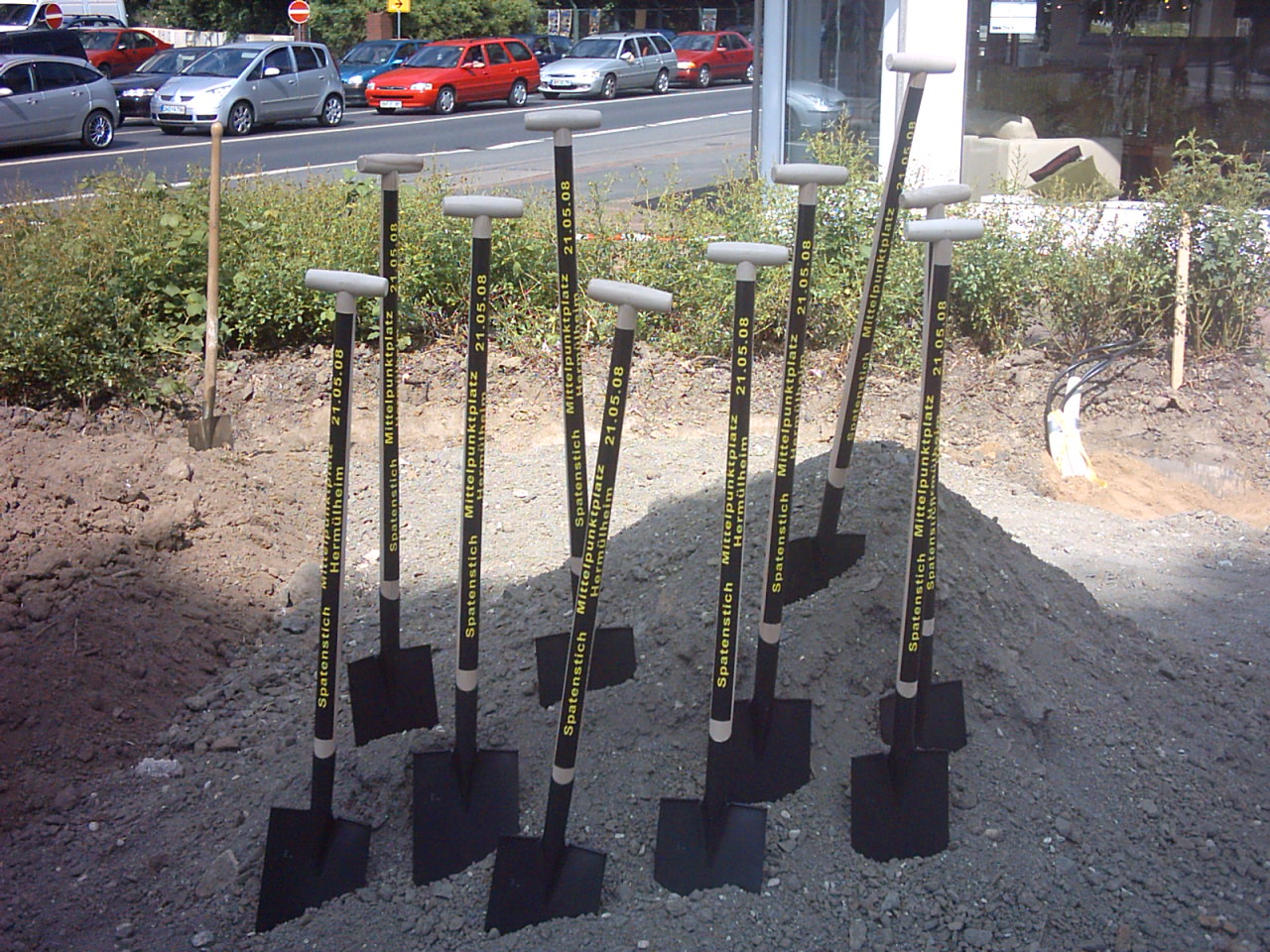The image depicts an outdoor scene featuring a pile of light grayish gravel intermixed with darker brown dirt. In the foreground, ten black metal shovels with black handles are prominently planted into the ground. Each handle is adorned with yellow writing, possibly indicating a company name in another language, suggesting these tools might be part of a groundbreaking ceremony. The handles culminate in thin, oval grips designed for two-handed use. Surrounding the gravel pile are sparse, taller shrubs and grasses. Further in the background, a busy highway with multiple cars moving in one direction is visible. To the right, there's an older wooden shovel embedded into the brown earth, alongside a building with an open window through which a sofa or couch is partially seen. This image captures a rich tapestry of elements, combining the anticipation of a new construction event with the everyday bustle of life in the background.